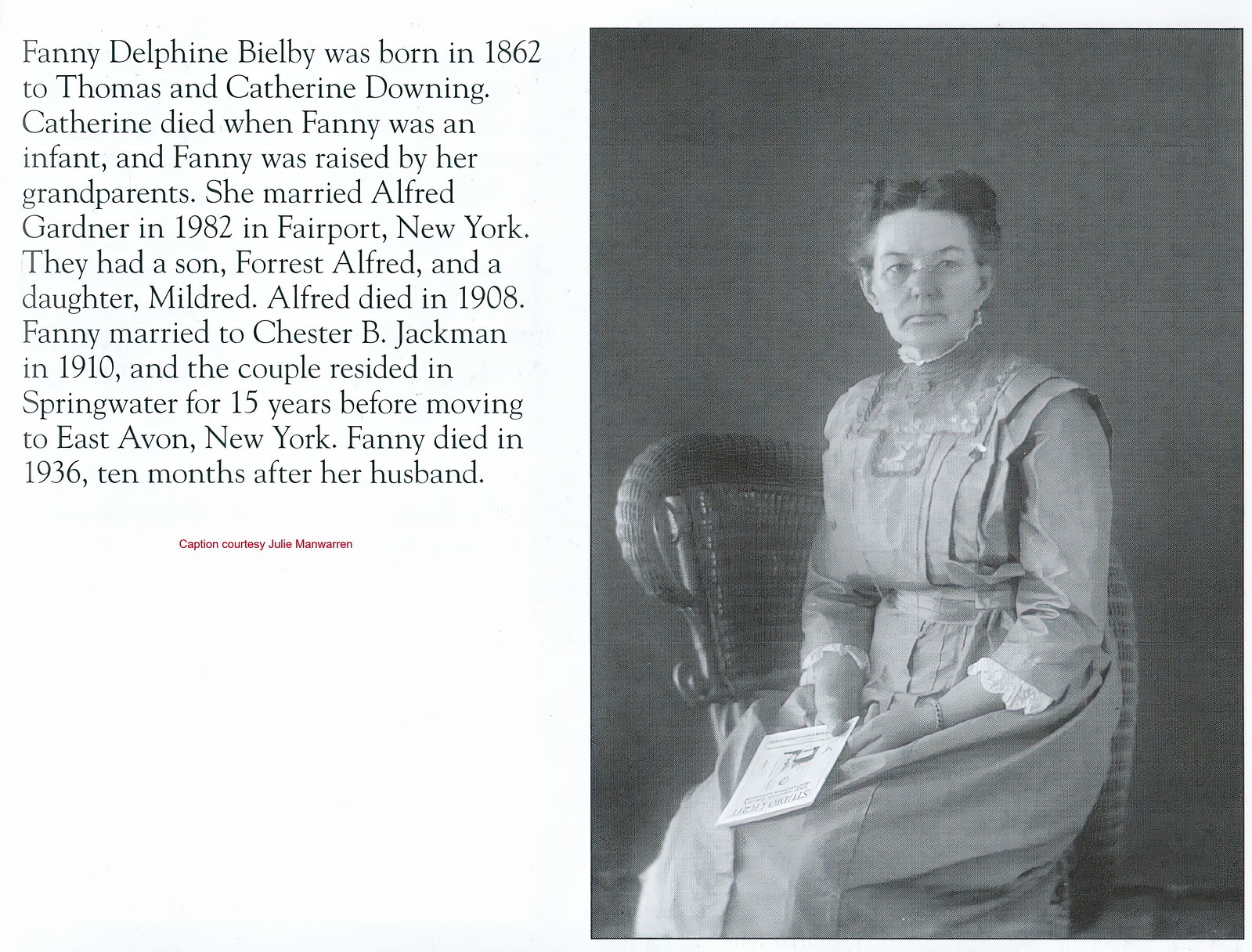The rectangular image is divided vertically, with a black and white photograph on the right side depicting a woman seated in a wicker chair, which features intricate curves and curls. The woman is dressed in a long, crinkled frock that has lace detail on the sleeves, and she holds a pamphlet in her hand while looking directly at the camera. On the left side of the image, there is an off-white background with gray text detailing the woman’s life. The text reads: "Fanny Delphine Bealby was born in 1862 to Thomas and Catherine Downing. Catherine died when Fanny was an infant, and Fanny was raised by her grandparents. She married Alfred Gardner in 1882 in Fairport, New York. They had a son, Forrest Alfred, and a daughter, Mildred. Alfred died in 1908. Fanny married Chester B. Jackman in 1910, and the couple resided in Springwater for 15 years before moving to East Avon, New York. Fanny died in 1936, 10 months after her husband.” The image, primarily in shades of black, white, and gray, serves as an informational piece about Fanny Delphine Bealby’s life and background.